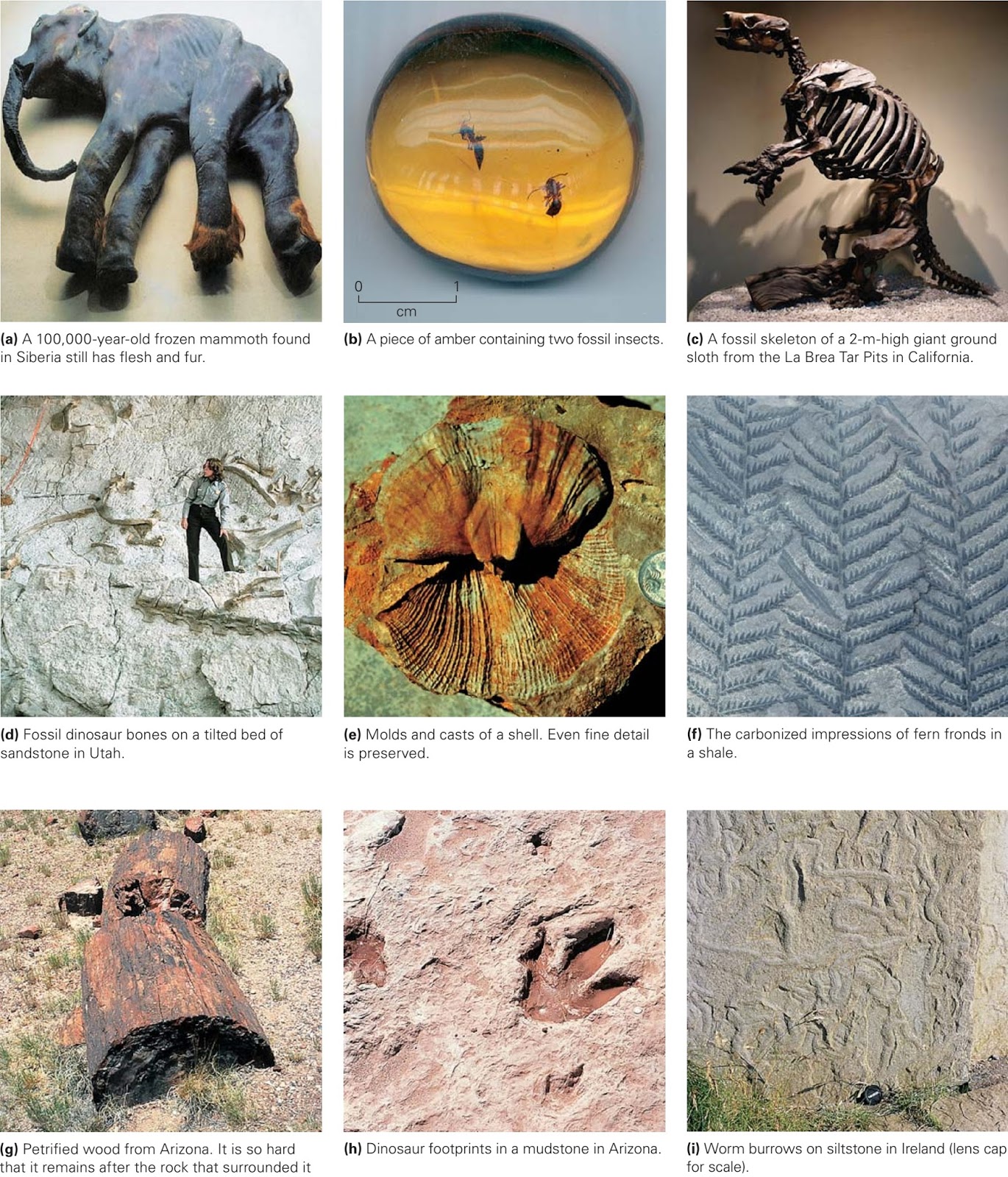The image is a large, square collage composed of nine smaller squares, each showcasing a different historical artifact, all labeled A through I with descriptive text beneath them. In the upper left corner (A), there's a statue-like figure of a mammoth lying on its side, described as a 100,000-year-old frozen mammoth found in Siberia, remarkably still having flesh and fur. To its right (B), there's a transparent piece of amber containing two fossilized insects. Further right (C) is a fossil skeleton of a two-meter-high giant ground sloth from the La Brea Tar Pits in California.

Moving to the second row, the first image (D) features fossilized dinosaur bones with a female archaeologist standing in the background. The middle image (E) shows molds and casts of a shell, with even the finest details preserved in vibrant orange and yellow colors. The last image in this row (F) is a detailed carbonized impression of fern fronds in a shell.

On the bottom row, the leftmost image (G) displays petrified wood from Arizona, with several pieces scattered on a grassy surface. The middle image (H) captures dinosaur footprints in mudstone from Arizona, resembling chicken feet imprints. The final image (I) shows worm burrows on siltstone from Ireland. The collage collectively presents a diverse array of geological and paleontological artifacts, emphasizing the variation in preservation and the wealth of historical information they offer, likely curated from a historical museum exhibit.